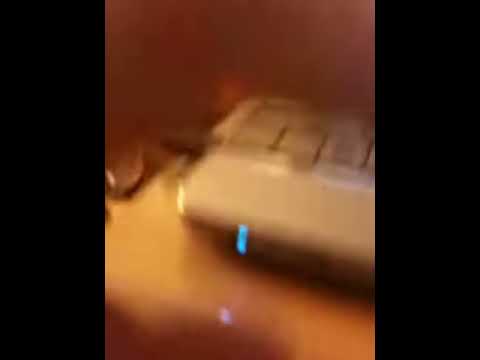The image features a very blurry and indistinct scene that is challenging to interpret clearly. A thick black border frames both the left and right edges of the picture, highlighting the blurriness of the central content. In the midsection of the image, a rectangular white object is visible, possibly a keyboard or a small electronic device with buttons on top. The device is emitting a faint blue light, indicating it is powered on. Partially obscuring the object, a hand is visible, adding a unique and relaxed element to the photo. The background reveals a hint of a wall at the top and a brown or yellowish wooden tabletop at the bottom, suggesting the setting is a casual, laid-back indoor environment. Despite the lack of clarity and the overall dark, reddish-brown tone, the image conveys a sense of a cool and unique design through its composition.